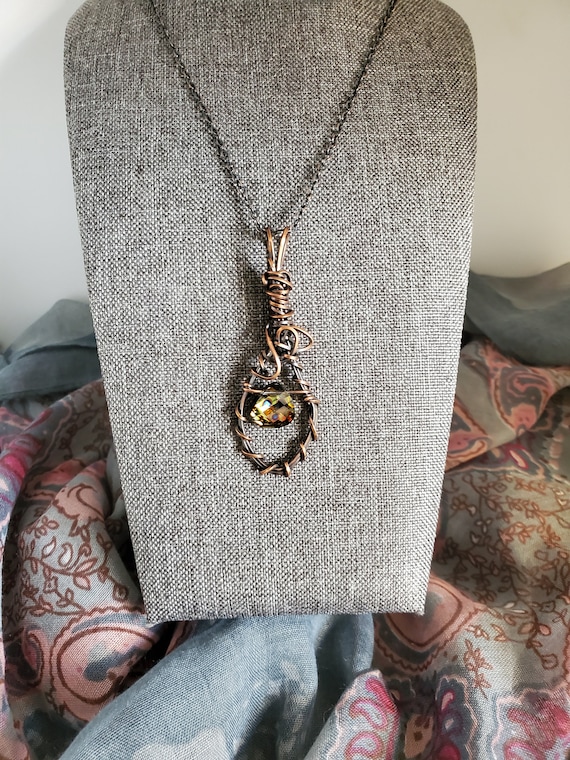This color photograph captures an intricately designed necklace as its focal point. The necklace features twisted copper and brass wires that form a looped pendant, showcasing a vibrant yellowish-gold gemstone, possibly citrine, at its center. The pendant is suspended from a thin silver chain, elegantly draping over a gray, canvas-like jewelry display board shaped to emulate the neck and décolletage. The background consists of a lively arrangement of fabrics, including a pair of jeans with bleach stains and a paisley floral print fabric, creating a dynamic scene with peaks and valleys of cloth folds. The fabric background, featuring shades of blue and pink, adds layers of texture and color contrast to the soft pastel studio lighting that bathes the entire setting.